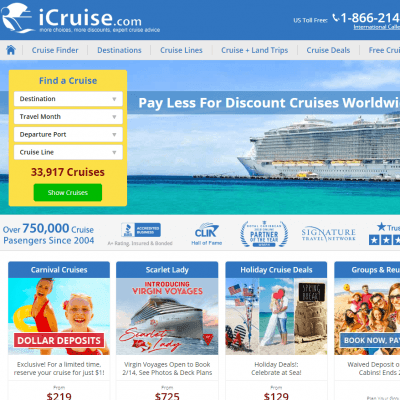**Detailed Caption:**

The image appears to be a screenshot from a webpage, likely a cruise booking site given the elements present. At the top of the page, there is a blue text box that features an icon of a cruise ship enclosed in a white circle. The cruise ship icon itself is blue. Adjacent to this icon, the text "iCruise.com" is displayed in white. To the right of this blue text box, white text reads "U.S. toll-free" followed by a phone icon and the number "1-866-214."

Directly beneath this top section is a gray text box containing several menu headers, each indicative of different browsing or booking options. The headers are labeled as follows: "Cruise Finder," "Destination," "Cruise Lines," "Cruise and Land Trips," "Cruise Deals," and "Free Cruises." On the far left of this gray text box, there is a blue home icon.

Below the navigation section, a large image of a cruise ship occupies considerable space on the left side of the page. The ship is set against a backdrop of aqua-colored water and a blue sky dotted with white clouds, giving a serene and inviting feel. To the left foreground of this image, a prominent yellow box serves as a search tool. This box allows users to find a cruise by searching via destination, travel month, departure port, and cruise line. Emphasized in red within this search area is the text "33,917 cruises." At the bottom of the yellow box, a blue button is labeled "Show Cruises."

Further down, there is another text box with a gray background, featuring blue fonts. This box proudly states that over 750,000 cruise passengers have been serviced since 1994 and lists a variety of rewards. 

At the end of the webpage, four smaller boxes provide additional information and deals, each with a specific focus. The boxes are labeled: "Carnival Cruises," "Scarlet Lady," "Holiday Cruise Deals," and "Cruise Returns," summarizing different touring options available at the bottom of the page.